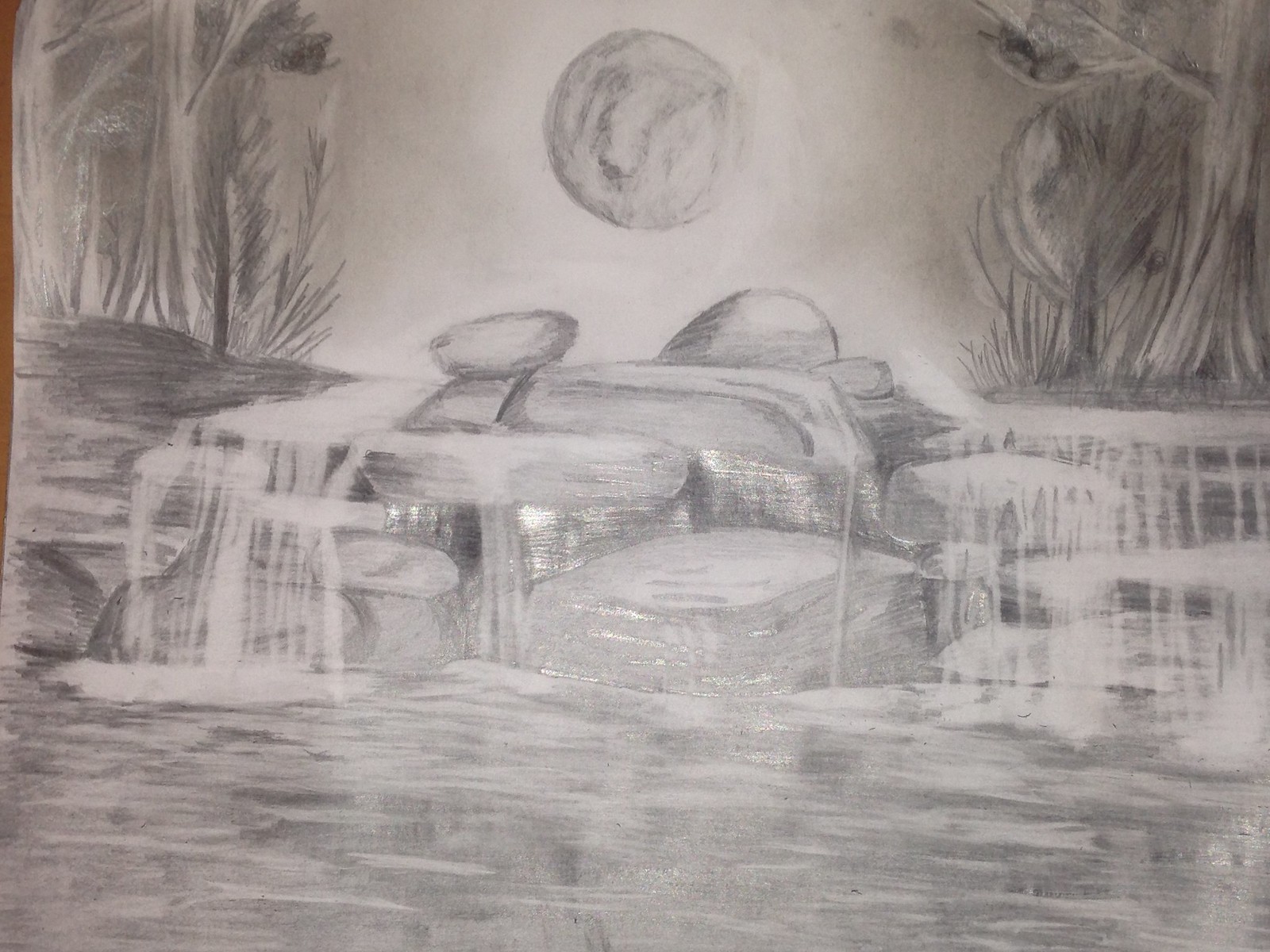A detailed pencil sketch depicts a serene outdoor scene centered around a tranquil pond and flowing stream. The monochromatic artwork, drawn meticulously in black and white, rests on a barely visible desk surface. In the foreground, smooth rocks form a cascading arrangement from which water appears to stream both left and right, creating a gentle, circular movement around a central point. The background is filled with tall, shadowy trees, giving depth to the composition. Around the stream, lush ferns and plant life add intricate details to the natural landscape. An ethereal light source in the sky, possibly representing either the moon or the sun, casts a soft glow over the scene, enhancing its tranquil and mysterious atmosphere.